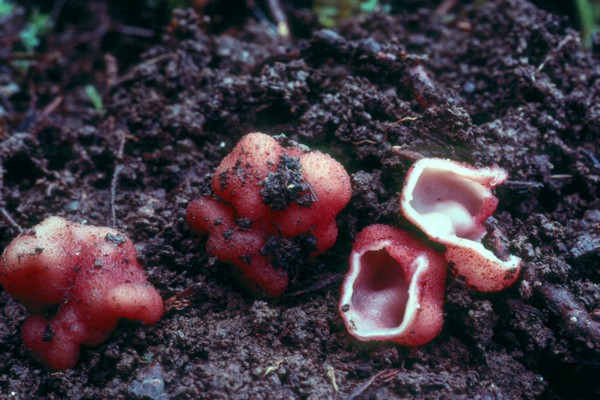The image is a close-up of dark, rich, and somewhat damp soil with scattered organic matter. Prominently featured are three reddish-pink, amorphous seed-like or fungi structures. In the upper part of the soil are small sprigs of green growth. The fungi have a peculiar texture, somewhat akin to fruit rinds or mushrooms. The one on the left-hand corner and the one in the center of the image are whole, while the one on the right is split open, revealing its pale pinkish-white interior. The halves of the broken fungi lie side by side, exposing the contrast between their vibrant outer shell and the lighter interior.